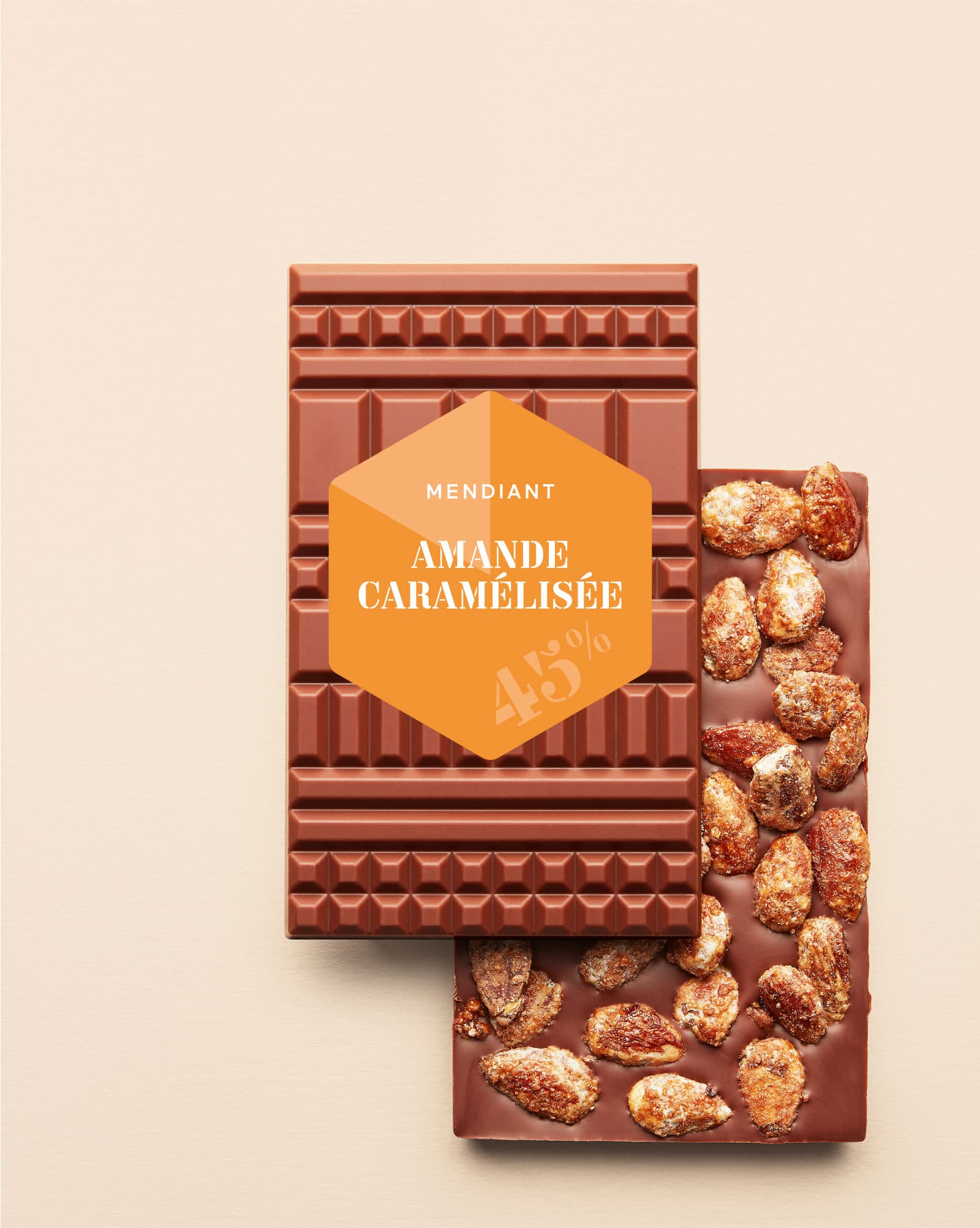This product image features two milk chocolate bars against a beige background. The primary chocolate bar on top showcases an intricate design of various rectangles—long, medium, and fat, creating a visually appealing geometric pattern. The front bar partially covers a second bar beneath it, with the bottom right corner of the second bar peeking out. This second bar appears turned backwards, displaying its textured backside, which is embedded with what seems to be roasted and spiced pumpkin seeds or perhaps candy-coated almonds. The chocolate's pattern contrasts with the partially visible back bar, where nuts sit atop the surface, suggesting they were added as the chocolate cooled.

Prominently placed on the top bar is a sticker in the form of an orange hexagon, containing product details in white text. It reads "Mendiant" at the top, followed by "Amande Caramelisée," and "45%" at the bottom. This label indicates the product name and specifics, with the geometric shapes on the packaging enhancing the 3D appearance. The entire setup is designed to highlight both the front and back textures of the chocolate, emphasizing not only its aesthetic appeal but also the embedded nuts, likely almonds, on the backside.